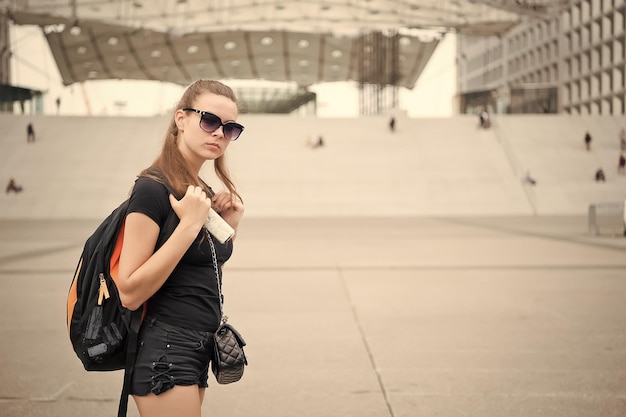This photograph captures a young woman, possibly in her late teens or early twenties, standing slightly to the left of center on a large, paved concrete area. Her long, dirty blonde to light brown hair cascades over her shoulders, and she is wearing large, dark sunglasses that obscure her eyes. She dons a black short-sleeved shirt and black shorts, highlighted by a pair of small zigzag strings on the sides. The woman carries a black backpack with orange accents and holds the straps with both hands, while a black quilted crossbody purse with a silver chain rests at her hip. She appears to be frowning or pursing her lips, giving her a slightly unhappy or contemplative expression. In her right hand, she clutches a white object, possibly a phone or some paper. 

The background features a significant incline with broad concrete steps, possibly part of a large plaza or public space, where people can be seen sitting and walking, though they are not the focal point and appear blurred. The steps are flanked by indistinct buildings; on one side there might be an office building extending upwards out of the frame. Some structures on top of the steps could be a canopy, stage, or museum entrance, contributing to the sense that this area is a bustling, open-air environment, perhaps frequented by tourists or visitors. The photograph, horizontally oriented and likely taken during daylight, shows some digital editing which adds to the slight visual surrealism.